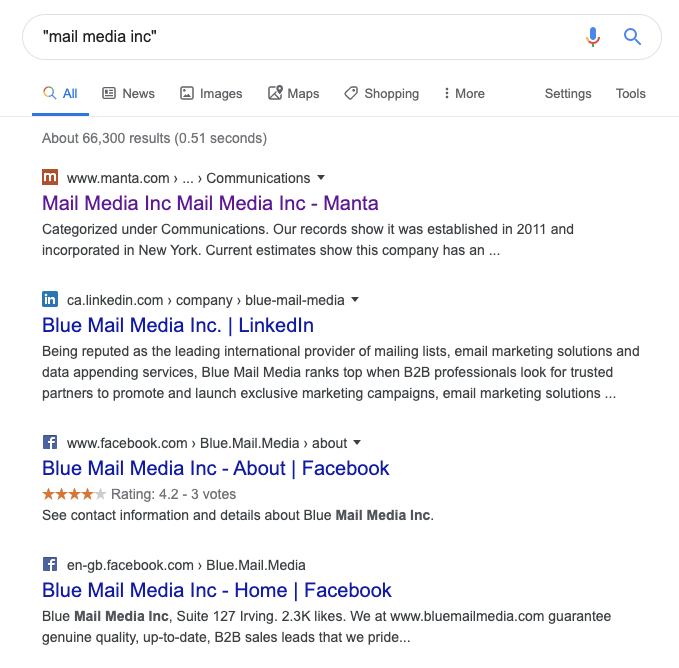**Detailed Caption:**

The image captures a screenshot of a Google search results page, though the Google logo is not visible. It clearly shows a user has searched for "Mail Media Inc." The search bar is prominently located at the top, accompanied by the microphone and magnifying glass icons on its right.

Below the search bar, there is a menu bar with various options, each marked with a respective icon: "All" (magnifying glass), "News" (newspaper), "Images" (picture), "Maps" (map), "Shopping" (price tag), and "More" (three dots). Further to the right are "Settings" and "Tools."

The search yielded approximately 66,300 results in 0.51 seconds. The first search result is from www.manta.com, detailing Mail Media Inc. under communications. It notes that the company was established in 2011 and incorporated in New York, though the text cuts off mid-sentence.

The next result, from ca.linkedin.com, describes Blue Mail Media Inc. It highlights the company's reputation as a leading international provider of mailing lists, email marketing solutions, and data appending services. It positions Blue Mail Media as a top choice for B2B professionals seeking trusted partners for exclusive marketing campaigns, though this description also ends abruptly.

Following that, the third result from www.facebook.com gives a brief overview of Blue Mail Media Inc. It mentions that the company has a rating of 4.2 stars from three votes and provides contact information and deals.

The fourth result from engb.facebook.com lists Blue Mail Media Inc.'s location at Suite 127 Irving, noting it has 2.3K likes. It assures genuine, up-to-date B2B sales leads through its website, bluemailmedia.com, though once again the description is incomplete.

Overall, the screenshot offers a detailed glimpse into search results for Mail Media Inc., prominently featuring related entities such as Blue Mail Media Inc. through various platforms including Manta, LinkedIn, and Facebook.